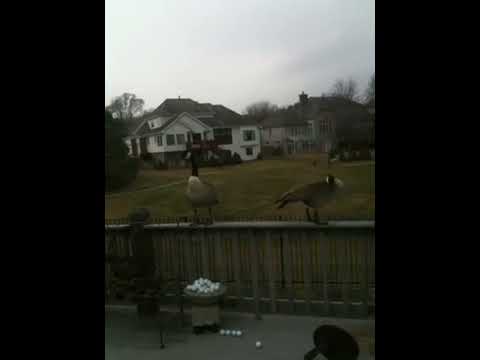The image captures an outdoor scene likely from a backyard or patio, looking outwards. In the foreground, there's a railing fence with two birds, possibly geese or ducks, perched on it. Below the fence, there appears to be a table or stand with several golf balls, and a few more balls scattered on the ground. The scene extends into a vast, well-maintained lawn leading to two large mansions in the distance—one painted white and the other brown. The setting is on a cloudy, overcast day, contributing to the muted tones of white, gray, dark gray, brown, green, and dark green visible in the image. The two birds are centrally positioned, drawing initial focus, framed by the expansive field and grand homes in the background. There are no text elements visible in the picture.